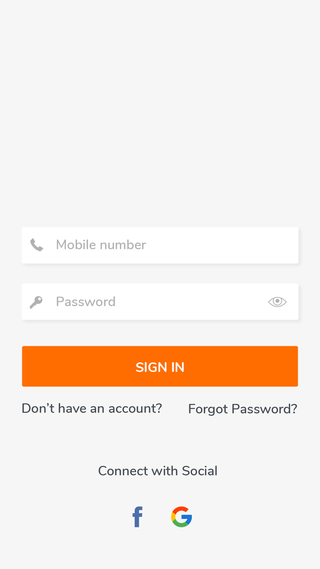The image depicts a minimalistic sign-in page for a mobile app, characterized by its vertical rectangular layout. Prominently centered in the design are two input fields: the first inviting users to enter their mobile number, and the second to input their password. Below these fields lies a conspicuous orange button with white text that reads "Sign In." 

Adjacent to this button are two ancillary options: "Don't have an account?" on the left, and "Forgot password?" on the right, catering to different user needs. Below these, the text "Connect with Social" suggests additional login methods, although the exact app remains unidentified. At the very bottom center, icons for Facebook and Google indicate that users can alternatively sign in using these social media accounts, providing flexibility and convenience.